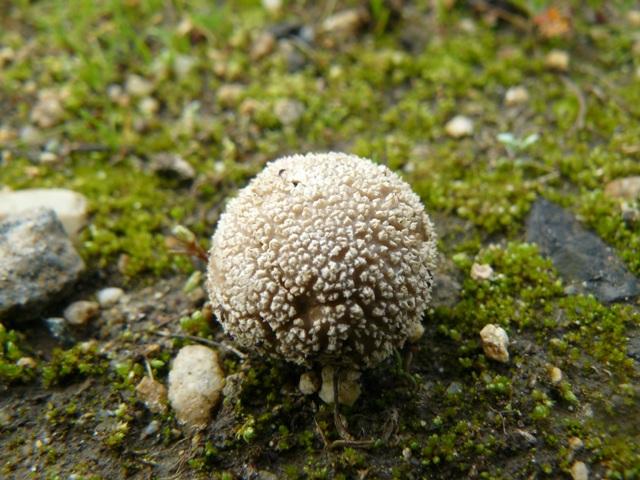The image depicts a damp, moss-covered ground abundant with various rocks and pebbles, displaying a range of colors including black, tan, and white. The foreground is in sharp focus, highlighting a round, globe-like object that appears to be a puffball mushroom. This centerpiece has a brown base with white, spiny protrusions giving it a texture similar to coral or shag carpet. The soil is visibly wet, suggesting a marshy or swampy environment. Surrounding the puffball are rocks of differing sizes, with the largest located to the left. The background of the image is blurry, but hints at an inclined hillside, possibly with tree roots or a tree stump, adding depth to the scene.